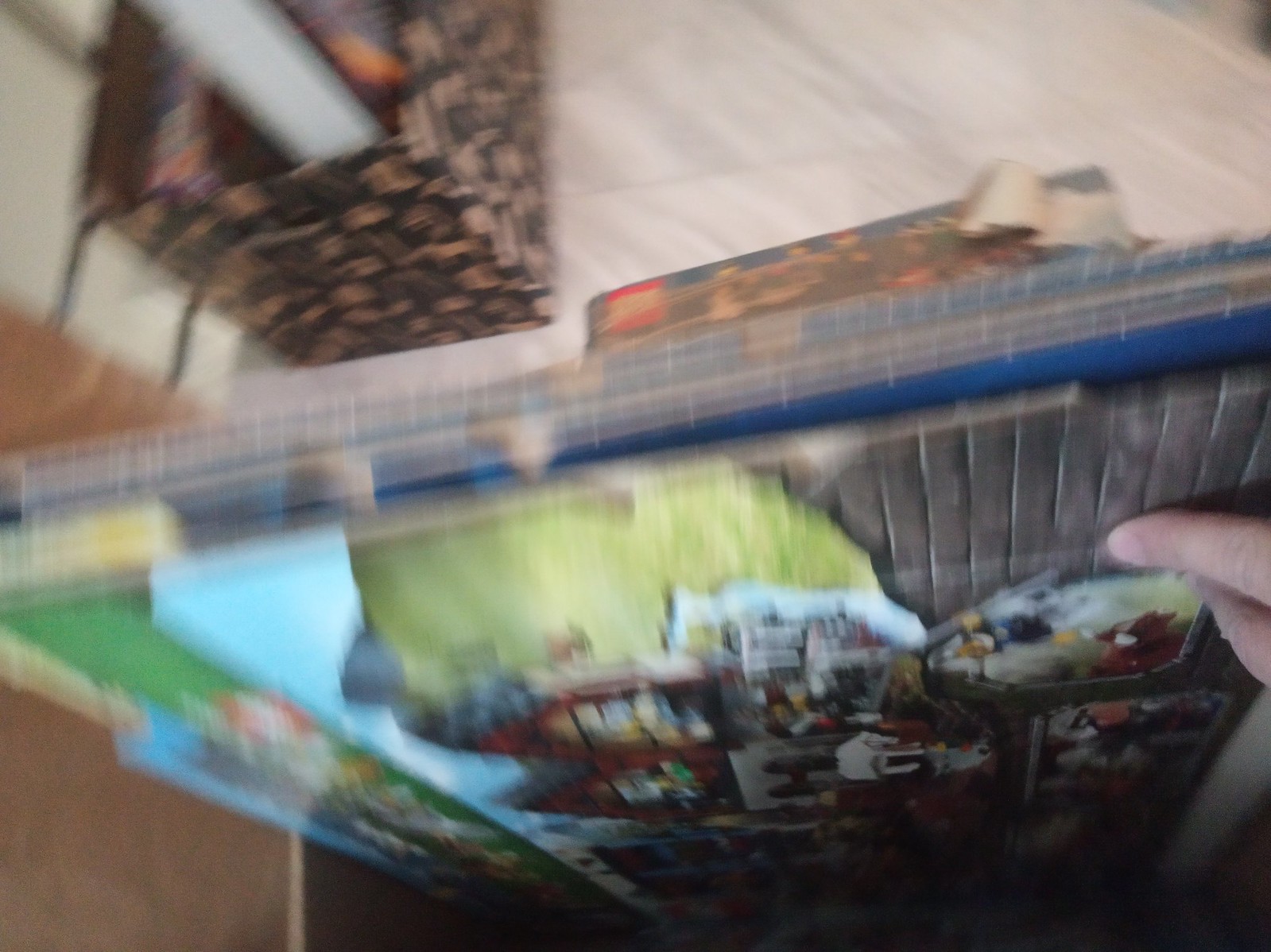In this very blurry photograph, we can make out a large rectangular wall decoration, possibly a poster, depicting a Christmas-themed house with multiple rooms. The image appears to have been taken with a fast-moving camera, causing everything to be out of focus. At the top of the photo, there is a white floor visible. Below the floor, a black rectangular bin adorned with gold animal designs is partially filled with objects. On the right side, a light-skinned hand and finger can be seen holding up the wall decoration. The central element of the decoration showcases several buildings or houses that appear to have their fronts removed, offering a clear view inside. Surrounding these buildings are walls resembling gray cement.